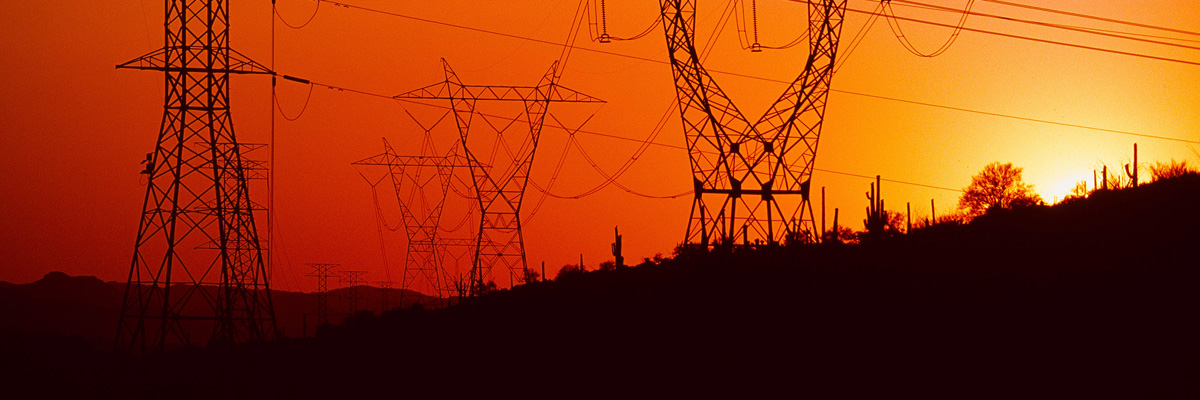The image captures an array of power lines stretching into the horizon, accentuated by the dramatic colors of a setting sun. There are four prominent power line structures, tall, black, and wiry, arranged in two parallel rows that recede into the distance, becoming less distinct as they blend into the horizon. The sky transforms from a vivid yellow near the sinking sun on the right side to a burnt orange on the left. This gradient of warm hues contrasts starkly with the silhouetted power lines and the darkened land below. The lower part of the image is enshrouded in shadows, rendering the landscape—comprising a grassy field with hints of cacti—indistinguishable. At the far end, the silhouette of a low mountain range or hills is faintly visible, accompanied by what appears to be a small, almost imperceptible fence separating the land from the area occupied by the power lines. The absence of people adds a sense of solitude and focus to the stark, industrial beauty of the scene.